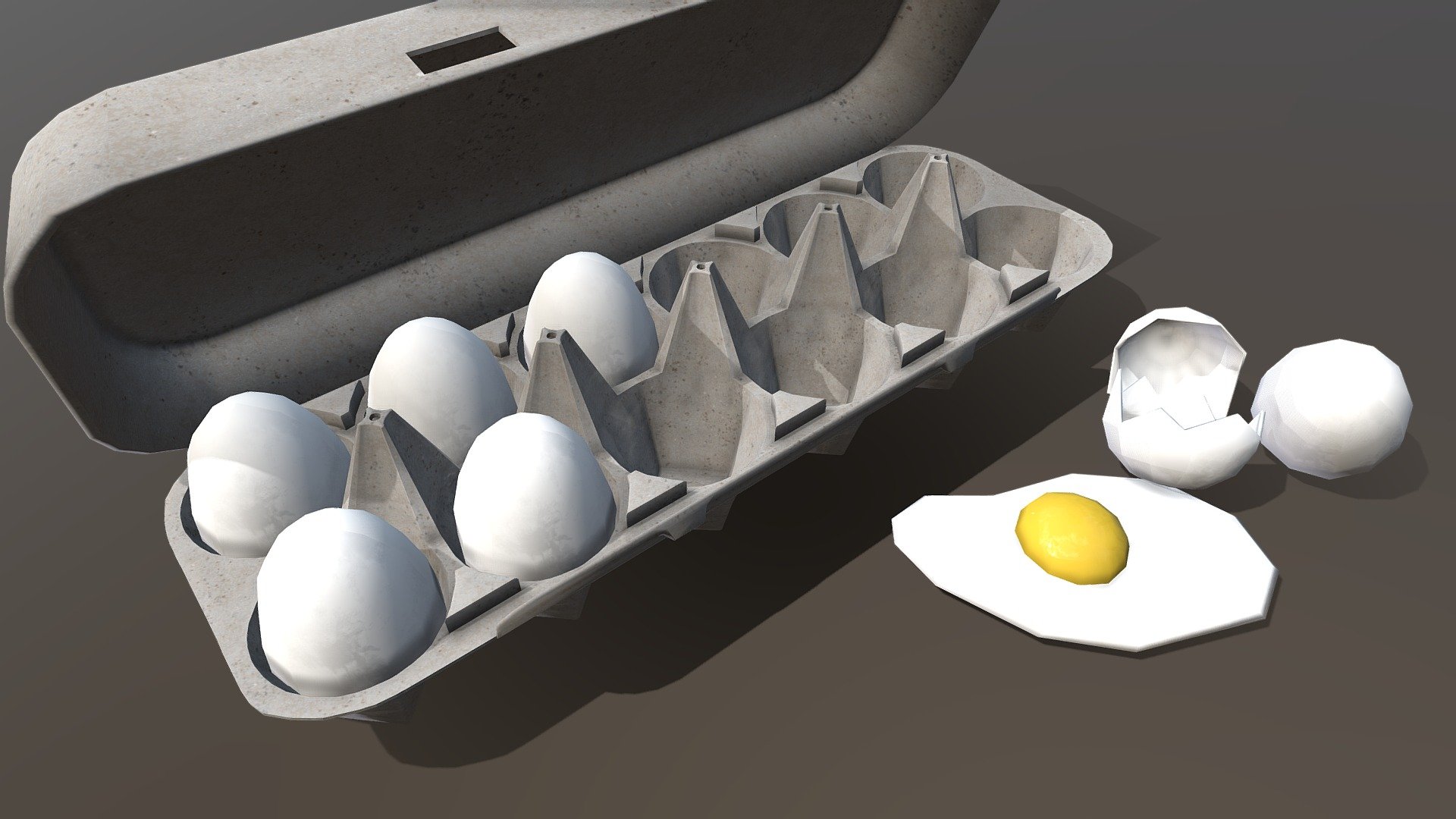The image is a color, computer-generated depiction of a gray 12-egg carton positioned in the upper left corner. The carton is open, revealing five eggs with a light white to grayish hue, while seven compartments are empty. Below the carton, to the front right, a separate whole egg lies outside, and nearby, a split eggshell reveals a fried egg with a distinct yellow yolk and white egg white. The entire scene is set on a grayish-brown background. The eggs, particularly the fried one, appear oddly angular with straight, choppy edges, diverging from the typical rounded shapes seen in reality. The lighting, which casts a shadow towards the lower left, suggests illumination from the upper left of the image.